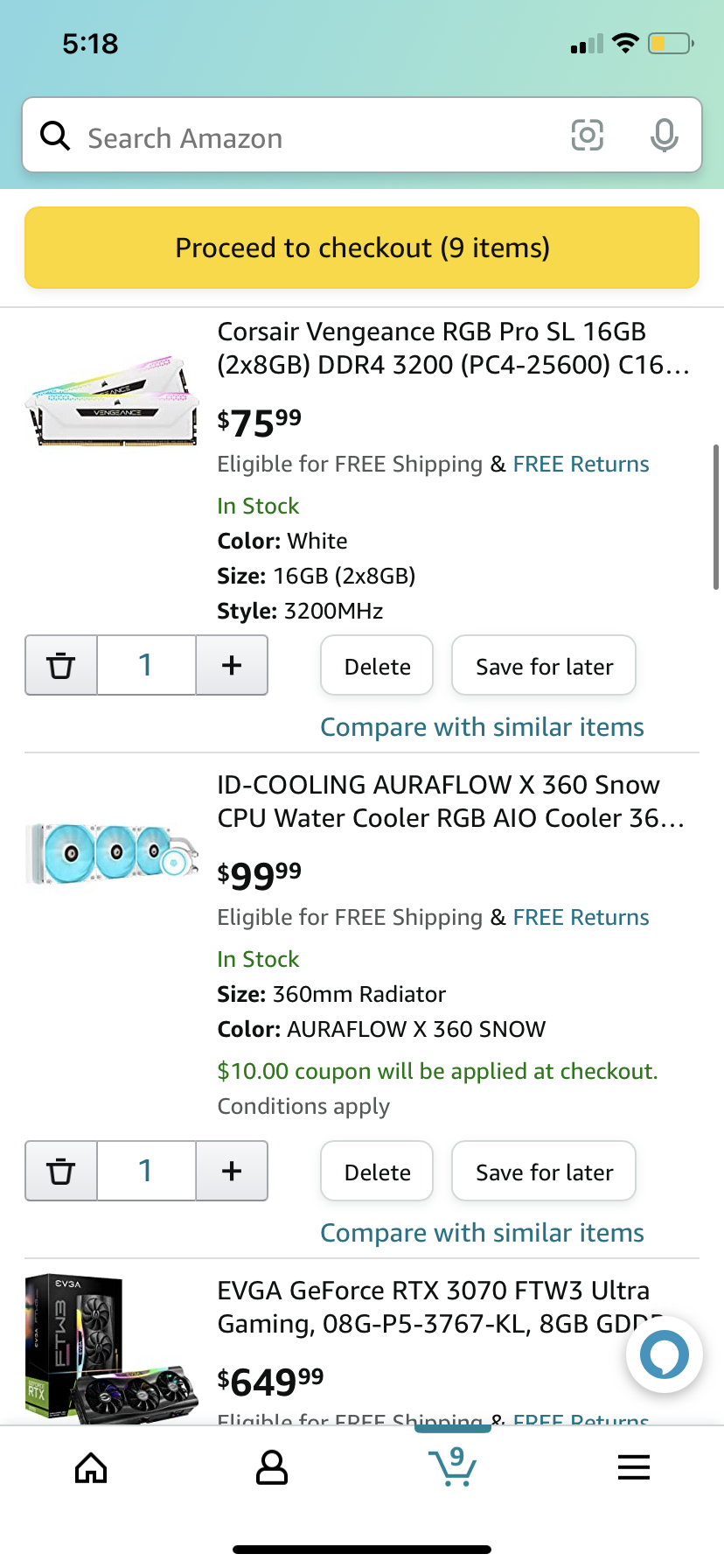The image features a digital shopping cart interface with a prominent green header against a white background, displaying the current time as 5:18. At the top of the page, there is a search bar, and beneath it, a yellow rectangle button labeled "Proceed to Checkout (0 items)".

The cart includes a detailed list of selected items:

1. **Corsair Vengeance RGB Pro SL 16GB (2x8GB) DDR4 3200 (PC4-25600) C16** - priced at $75.99 with the quantity set to one. This entry is accompanied by a "Delete" button, a "Save for later" option, and a blue link for "Compare with similar items".

2. **ID-COOLING AuraFlow X 360 Snow CPU Water Cooler RGB AIO Cooler** - listed at $99.99.

Each item title appears fully capitalized, showcasing the technical specifications and pricing clearly.